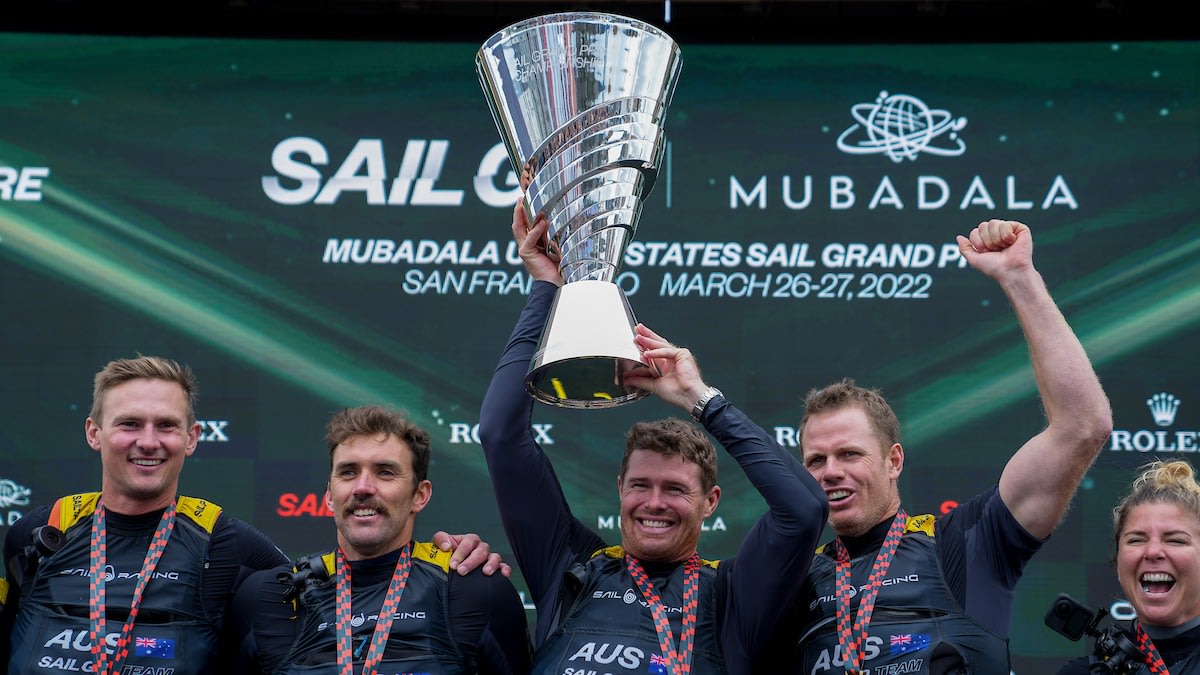The photograph depicts a jubilant celebration of an Australian sailing team at the Mubadala United States Sail Grand Prix held in San Francisco on March 26-27, 2022. Positioned against an emerald green banner with white text detailing the event, the image captures four men and a woman, all smiling triumphantly. The central figure, prominently displaying a large silver trophy with a conical shape, is flanked by teammates who sport black and blue uniforms adorned with "AUS" and the Australian flag. Each team member wears a red and blue lanyard, presumably attached to medals. The woman, situated on the right, with blonde hair and a broad smile, adds to the victorious atmosphere. The text in the background highlights the event specifics, including "SAIL G Mubadala," and sponsors like "Rolex," adding context to the team's grand achievement.